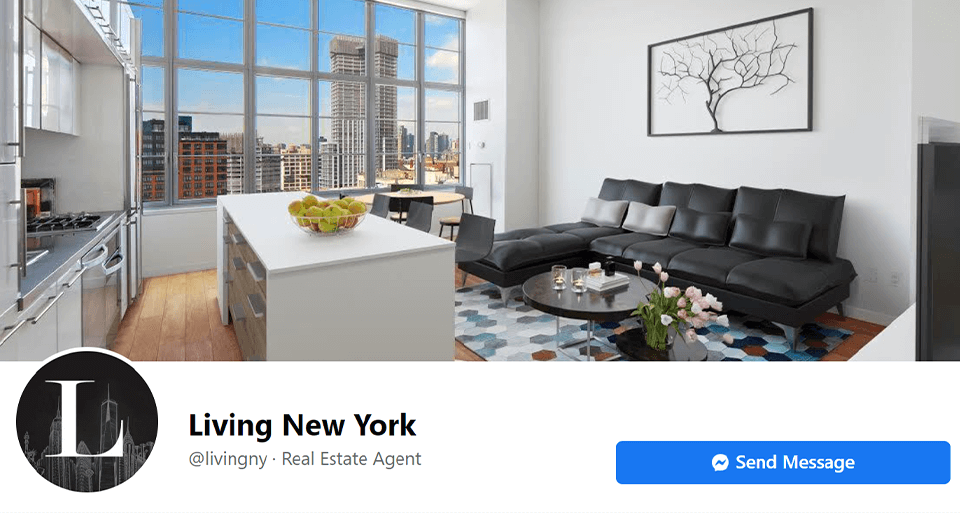A detailed caption for this image could be:

"This image is a screenshot of a section from a Facebook page showcasing a luxury apartment. The banner at the top of the page reveals the interior of an opulent living space, characterized by light gray walls adorned with a stylish black-bordered painting of a tree on a white background. The spacious room features a sleek black couch, beautifully accentuated with numerous cushions. A circular coffee table in front holds a couple of glasses and other small items, adding to the room's lived-in charm. Nearby, a smaller side table is adorned with a bouquet of vibrant pink roses. The apartment's modern kitchen area boasts a pristine white island topped with a bowl of fresh green apples. The stainless steel appliances, including the stove and refrigerator, enhance the contemporary aesthetics of the space. Beneath the image, black text reads 'Living New York, @Living NY, real estate agent,' accompanied by a black circular logo with a prominent white 'L.' To the right, a noticeable blue button inscribed with 'Send Message' in white invites viewers to engage further.”